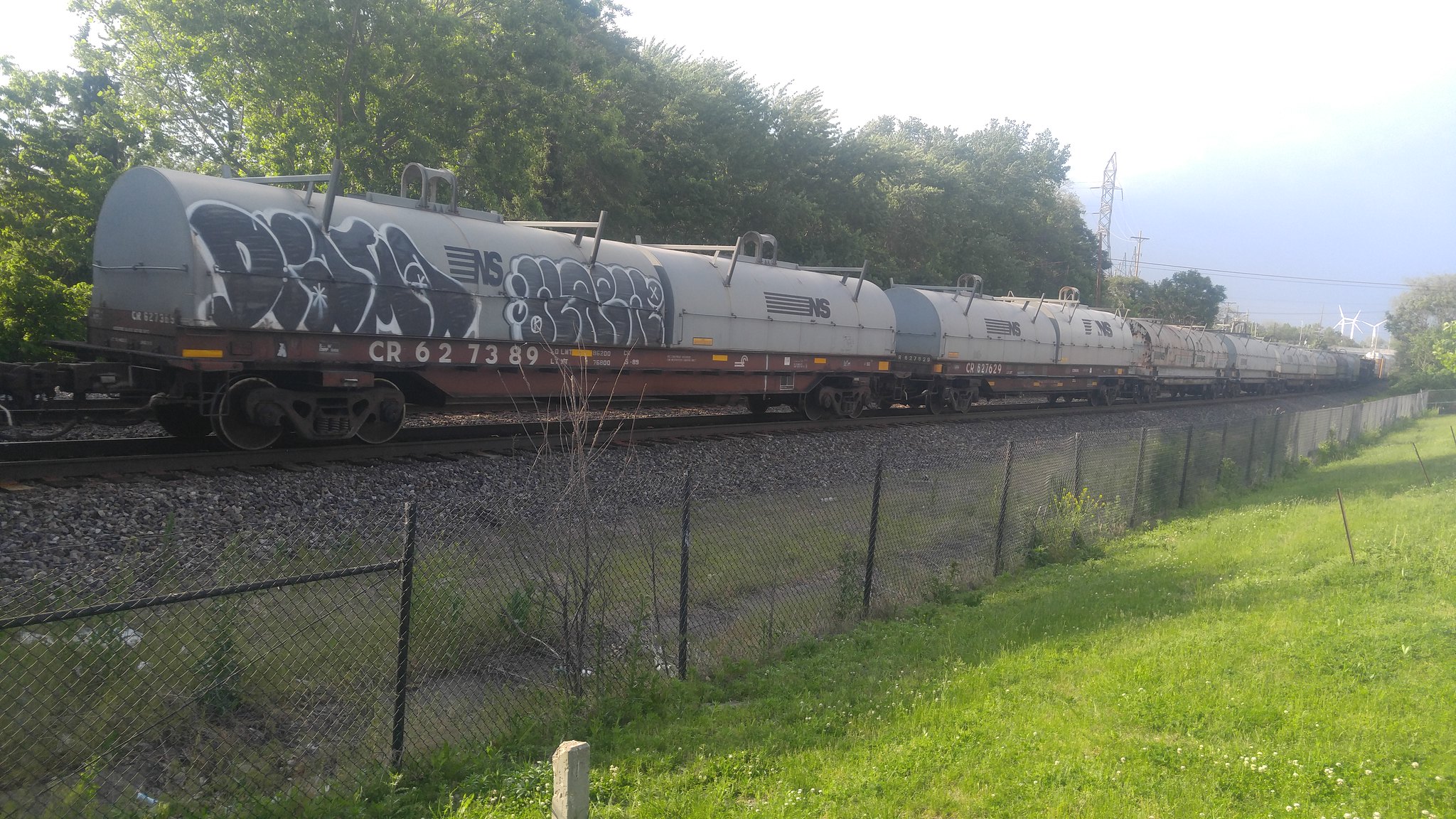The photo depicts a gray tanker train, identified by the number CR627389, situated on a railroad track amidst a scenic outdoor setting. The sky above is predominantly blue with patches of white clouds, adding to the tranquil atmosphere. To the left, a line of trees extends along the track, while a field of green grass bathed in sunlight dominates the right-hand side of the image, separated from the track by a chain link fence. The train itself appears to be carrying some type of liquid in its multiple tankers, probably four or five in number. Each tanker is heavily marked with graffiti, featuring large black letters outlined in white, though the exact words are unreadable. The rocky bed of the track is clearly visible in the foreground, and power lines run into the distance. A pole stands out in the middle of the composition, contributing to the overall balance of natural and man-made elements.